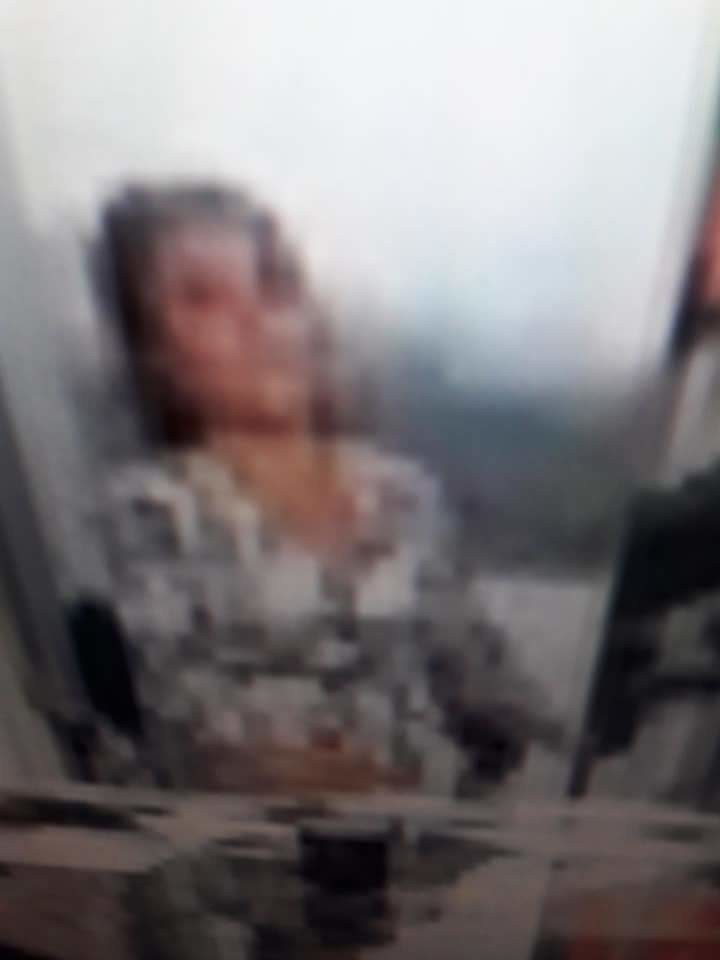This image depicts a blurred photograph of a woman or young girl seated at what seems to be a desk. She is dressed in a v-neck top adorned with a black and white geometric print. Although her face is indistinct, her dark, medium-length hair is clearly visible. The setting suggests she could be sitting in front of a screen, as her focus appears directed in that direction. A window behind her, draped with a white curtain, allows natural light to filter through, illuminating the scene softly. On the desk in front of her, various objects are scattered, though their exact nature is unclear due to the photo's blurred quality. The composition of the image gives a sense of a quiet, introspective moment captured in a homely environment.